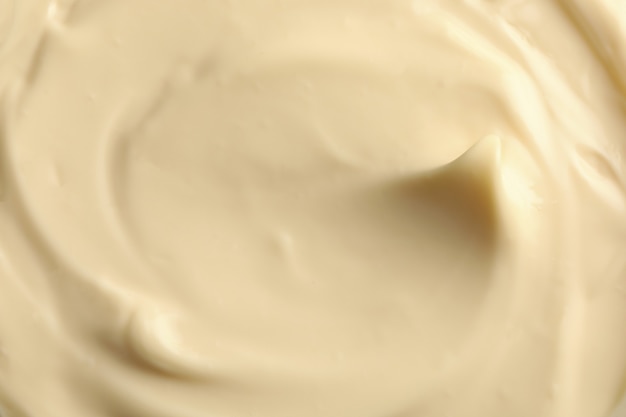The photograph is a close-up image of a thick, creamy white substance, occupying the entire frame with no visible background or container. The creamy material is comparable to mayonnaise, icing, or frosting, indicated by its highly opaque, viscous texture. The white cream appears smooth with subtle swirling patterns, and there's a noticeable peak or upward protuberance towards the center-right, suggesting it was manipulated by a spoon or a similar utensil. Light is shining from the upper right, creating a reflection and casting a shadow behind the peak. The substance has a slight creamy yellow tint, adding to its rich, dairy-like appearance.